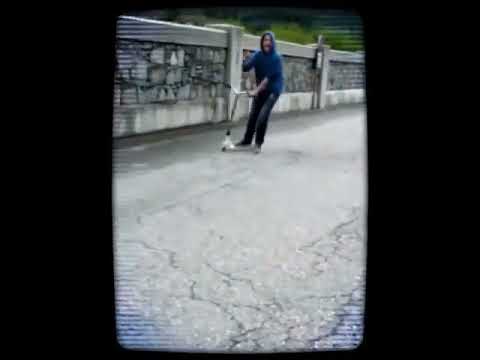This image, styled with rounded edges and scan lines reminiscent of an old CRTV screen, vividly captures a man on a silver, chrome-colored scooter with a black handle. The setup suggests a portrait mode focus. Dressed in a blue hoodie with the hood pulled over his head, black pants, and black shoes, the man stands with one foot on the scooter and the other foot on a cracked, weathered asphalt pavement. He has a brown mustache and dark hair, appearing to be in his mid-thirties.

The scene is set against a tall, imposing stone wall that runs behind him, composed of gray rocks and concrete with regularly spaced pillars. The bottom and top sections of the wall are reinforced with concrete, lending a sense of durability to the otherwise ancient-looking barrier. Three sections of this wall are prominently visible. 

Above this barrier, the blurred outlines of green trees are just discernible, suggesting the presence of nature beyond the concrete structure. The backdrop beyond the man fades into blackness on either side, further focusing the attention on the central figure and enhancing the retro aesthetic of the image.